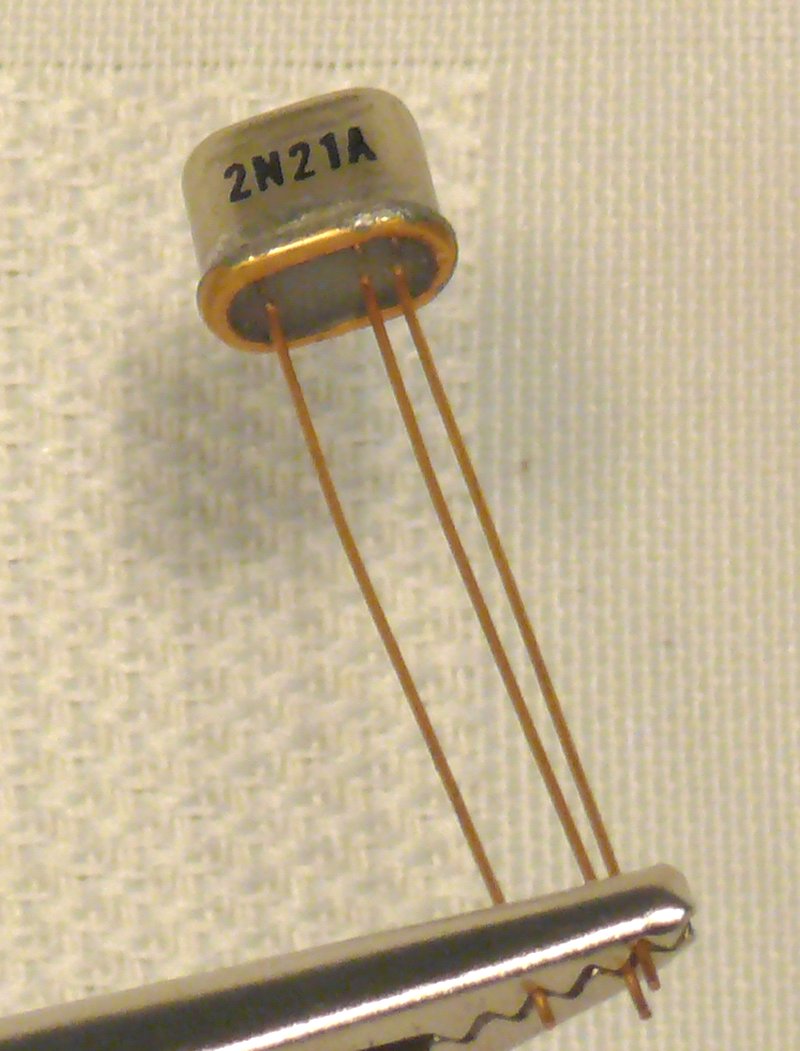This photograph features an extreme close-up of a small electrical component, precisely centered in the frame against an off-white, woven fabric background, possibly a napkin or placemat. The main subject is a single battery type capacitor, characterized by a small, metal, pot-like structure sealed with copper around its rim and labeled with the number 2N21A on its side. Extending from the bottom of the capacitor are three rigid, identical-length metal rods, likely made of copper. The rods are positioned with one on the left side and two on the right, appearing ready to be cut by a pair of wire cutters visible at the bottom of the image. These normal-sized tweezers, emphasizing the tiny scale of the capacitor, suggest its use in electronic circuit boards. The detailed close-up highlights the intricate design and potential utility of this essential electronic component.